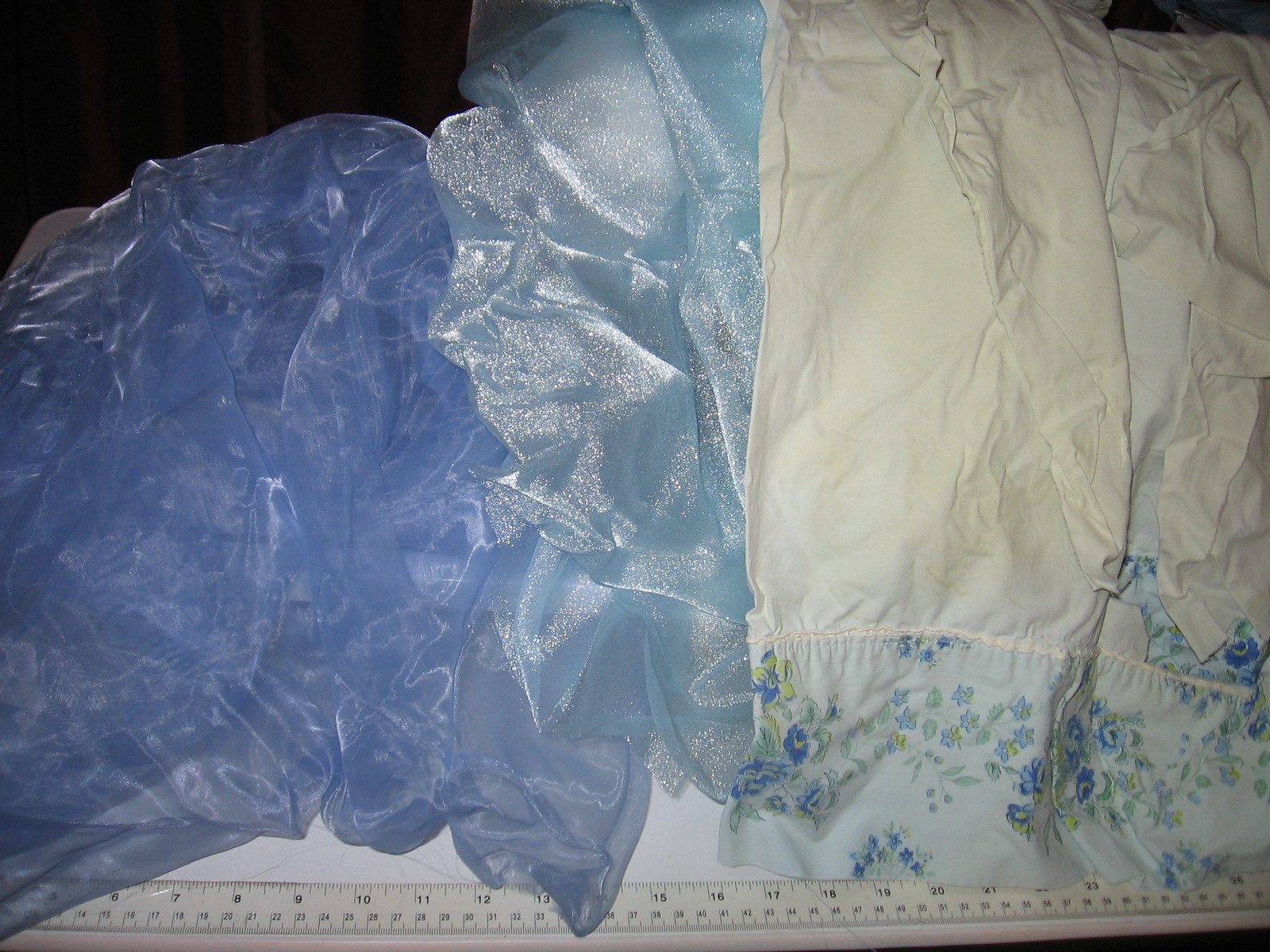This image features a detailed arrangement of various fabrics laid out on a white surface. At the bottom, there is a white or clear yardstick, displaying measurements in both inches (ranging from 6 to 26) and centimeters. Above the yardstick, on the left, rests a crumpled piece of light blue, almost see-through, shiny fabric, possibly chiffon or silk. In the center, there is another piece of blue, slightly iridescent material, also crumpled and similar in texture. To the right, there is a piece of white cotton fabric, possibly a pillowcase, featuring intricate blue fringes and decorated with small blue flowers. These fabrics are meticulously positioned, showcasing their textures and colors against the backdrop of the measuring tape.